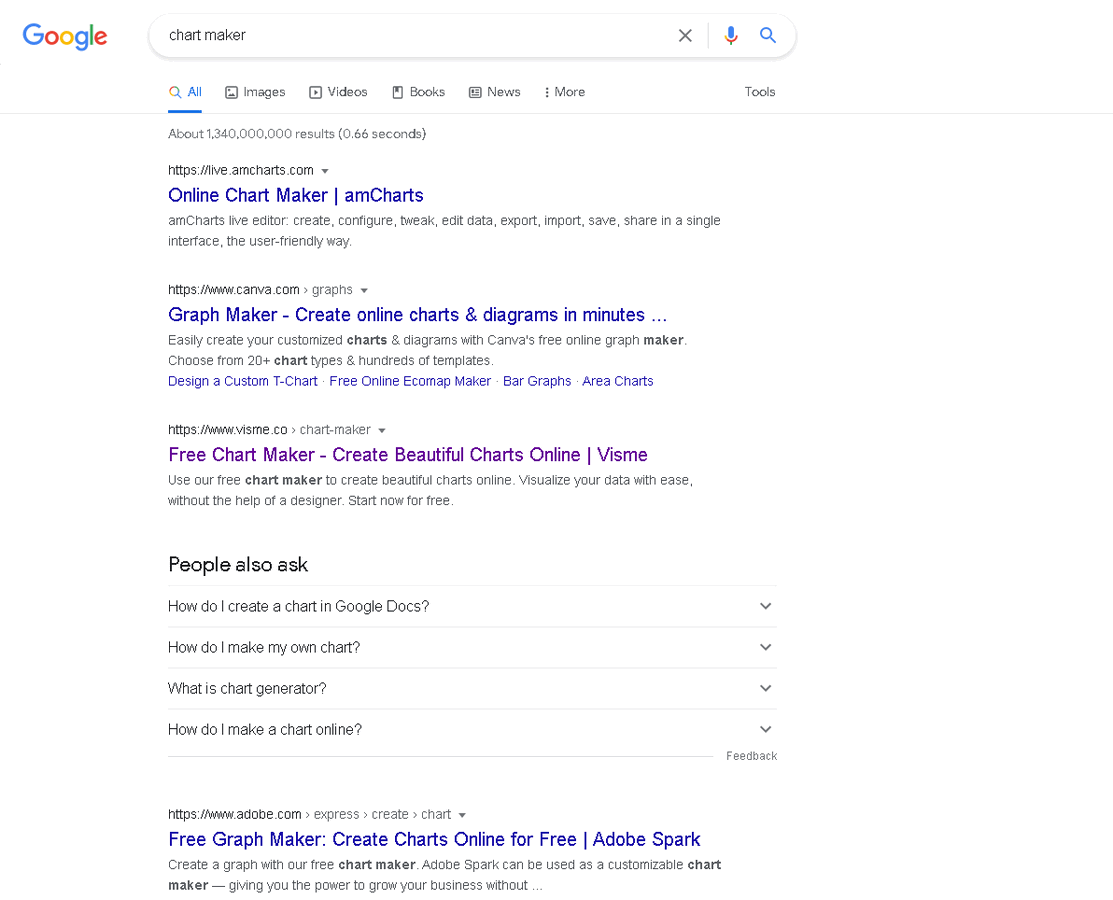This is a detailed view of a Google search results page for the query "ChartMaker". At the top, the iconic Google logo is prominently displayed, followed by the search bar containing the term "ChartMaker". To the right of the search bar are a closeout button (X), a Google microphone icon for voice search, and a magnifying glass icon for initiating the search. 

Directly beneath the search bar is a row of navigational tabs, including "All," "Images," "Videos," "Books," "News," "More," and "Tools" at the far right. These tabs allow users to refine their search.

The search results are listed in descending order. The top results include:
- "Online ChartMaker" 
- "AmCharts" 
- "GraphMaker - Create Online Charts and Diagrams in Minutes" 
- "FreeChartMaker - Create Beautiful Charts Online, Visme" (Notably, the link to Visme has been clicked.)

Further down the page, a section titled "People Also Ask" contains frequently asked questions within expandable boxes, each with a drop-down arrow on the right. These questions are:
- How do I create a chart in Google Docs?
- How do I make my own chart?
- What is a chart generator?
- How do I make a chart online?

The final search result at the bottom of the page highlights:
- "Adobe.com Express - Create Chart"
- "FreeGraphMaker - Create Charts Online for Free, Adobe Spark". 

Once again, this is a search results page generated from a Google search for "ChartMaker", with a clicked link labeled "FreeChartMaker - Create Beautiful Charts Online, Visme".